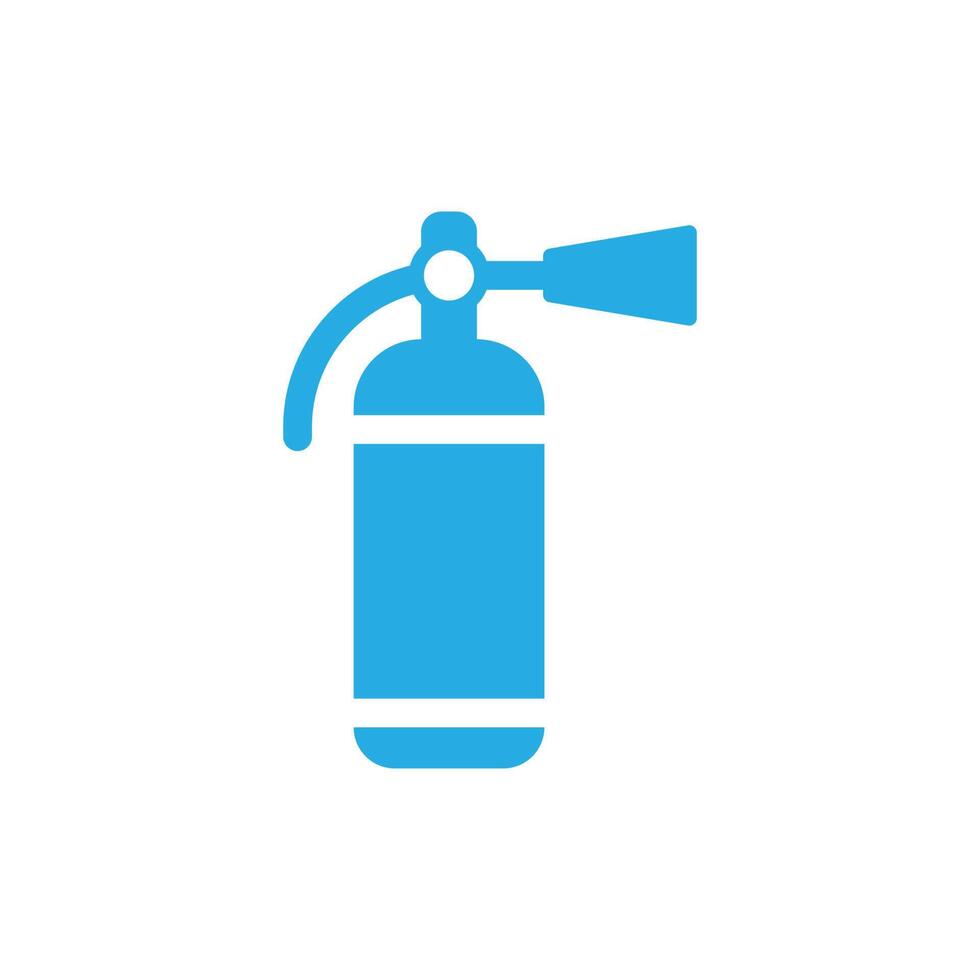This image features a light blue clip art drawing of a fire extinguisher set against a pure white background. The extinguisher has a cylindrical body with two horizontal white stripes, one positioned near the top and the other near the bottom, creating a segmented appearance. At the top of the extinguisher, there is a prominent white circle. Extending from the handle on the top left, a hose curves to the left and emerges on the right side, capped with a larger blue nozzle. The simplified vector design emphasizes the extinguisher’s key components without any accompanying text, ensuring the viewer's attention is solely on the detailed yet simplistic representation of the fire extinguisher.